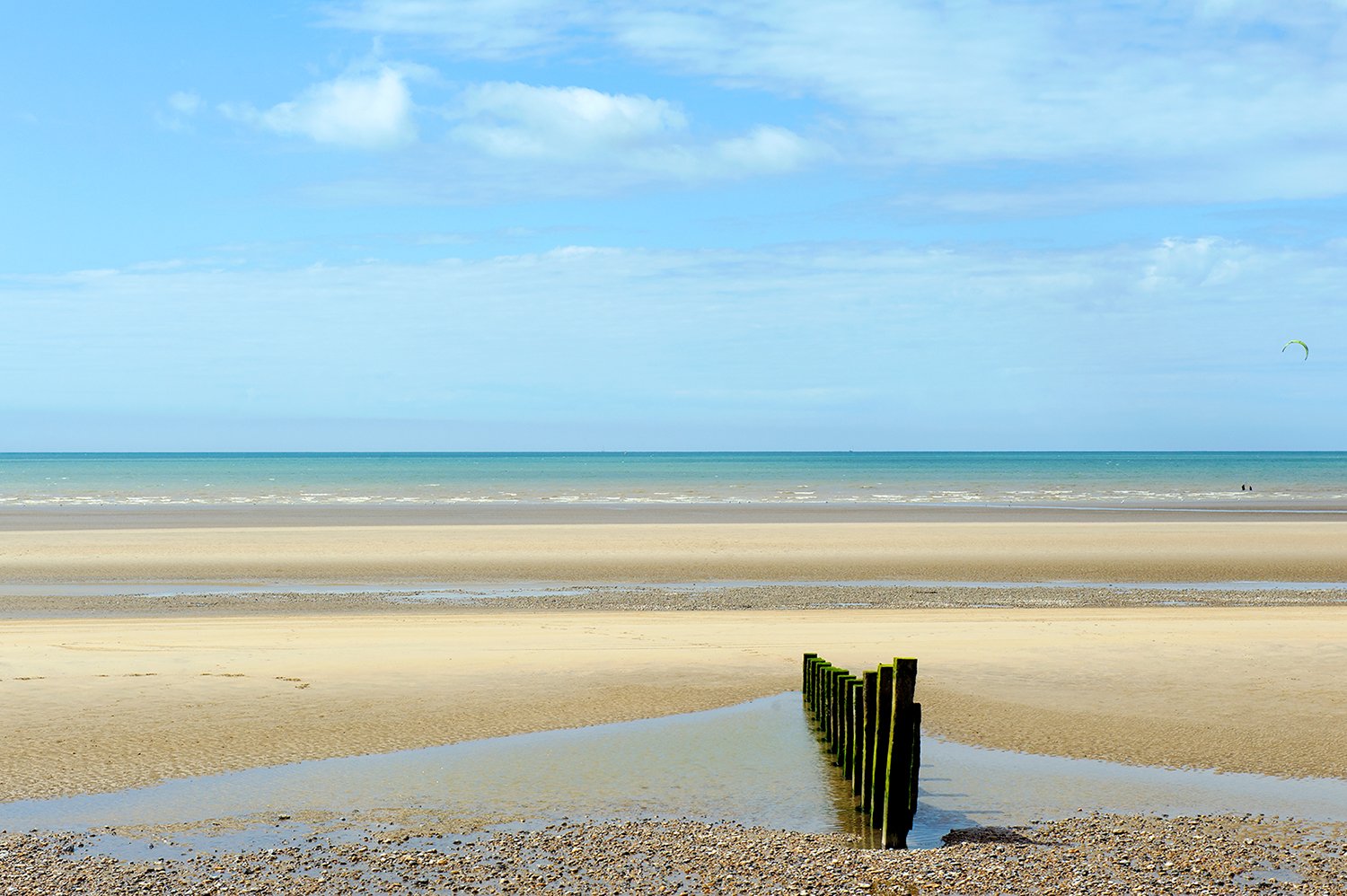This outdoor daylight color photograph captures a deserted beach scene with intricate details. In the foreground, an area of wet sand and pebbles is punctuated by a row of wooden logs or green posts, seemingly embedded into the ground. These posts, about 15 in number, are located in shallow, standing water within a small depression on the beach. Approximately 20 feet further towards the sea, another strip of wet sand is visible. Beyond this, the beach transitions into a long expanse of dry, light brown, and yellow sand leading up to the surf. The ocean stretches out in the distance, displaying a deep blue, crystal-clear expanse. On the horizon, two small black dots, possibly people, can be seen near the surf, one accompanied by what appears to be a kite or sail in the sky above them. The sky itself is a powder blue with sporadic, thin, wispy white clouds scattered throughout. The entire scene exudes a serene, desolate beauty, highlighting the natural elements of sand, water, and sky in harmonious detail.